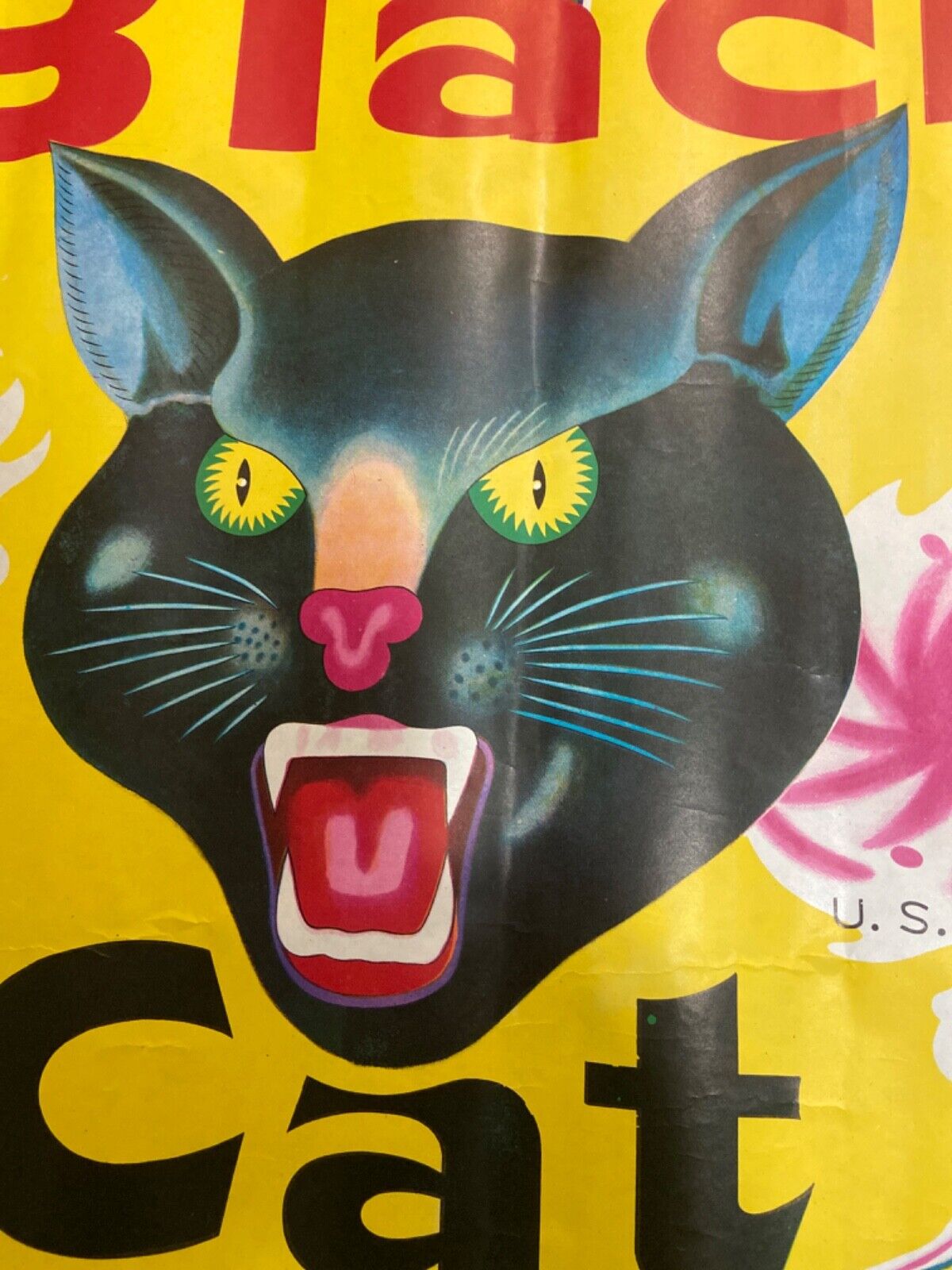The image is a vivid poster resembling a magazine cover, prominently featuring the face of a large, menacing black panther drawn in a cartoon style. The background is a striking bright yellow. The panther's head and face are the focal points, highlighted with a blue pencil shading that adds depth and dimension. Its ears are black with light blue interiors, and its whiskers are a vibrant neon blue. The panther’s eyes are intense, with bright yellow irises outlined in green, and narrow vertical pupils. The nose is a pinkish color, and its mouth is open, revealing sharp white fangs and a red tongue, giving it a ferocious, snarling expression. Surrounding the cat's face, partially visible bold red letters spell out "Black," while below, bold black letters spell out "Cat," though some of the letters are cut off. Additionally, there is a white circle mid-poster with a red spiral design inside and the letters "U.S." in narrow black text beneath it.